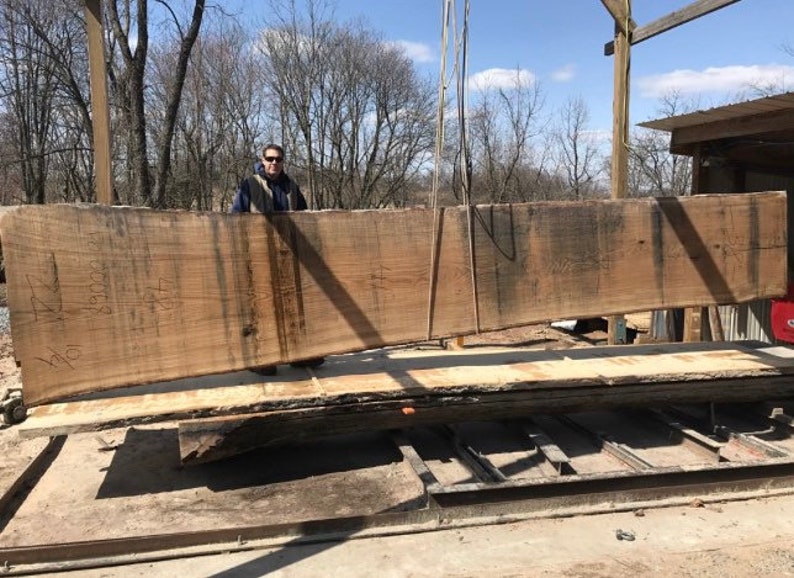The photograph captures a man standing behind a massive horizontal slice of a tree trunk, which is being suspended by ropes. The trunk slice, showcasing its age with its considerable width, hangs above a piece of machinery that is likely used for milling purposes inside a nearby building situated on the right side of the image. The suspension system is supported by a standing frame, with the trunk hovering over a set of steel rails laid out in a large rectangular frame, designed to bear the weight of such hefty items.

In the distance, several leafless trees can be seen, suggesting the season is either autumn or winter. The sky above is a clear blue adorned with a few scattered white clouds. The man positioned behind the tree trunk slice wears a dark top, has short dark hair, and sports sunglasses, adding a modern touch to this scene of industrial and natural elements. The ground beneath him is a sandy beige, contrasting the earthy tones of the tree trunk and the metallic sheen of the machinery.